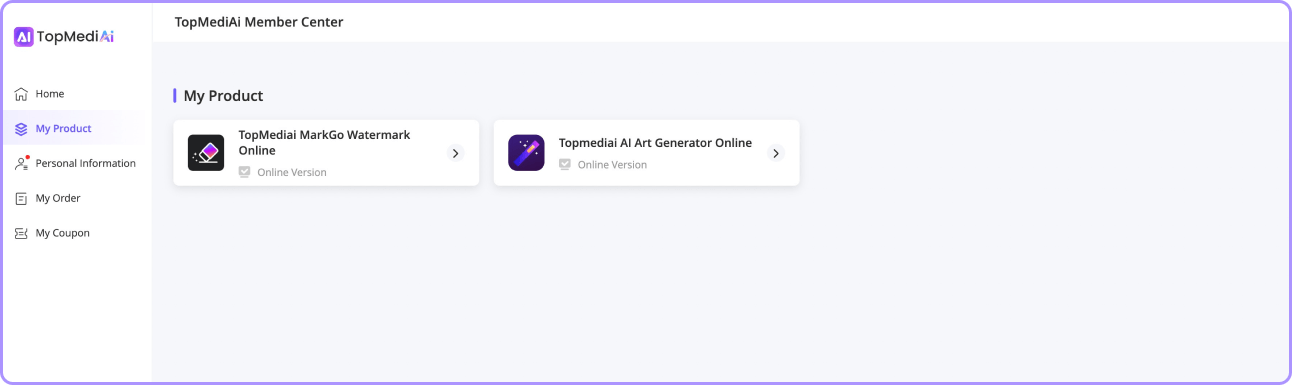This screenshot showcases the user interface of the website "Topmedia.ai," prominently displaying the "Member Center" at the top-left corner. The logo to the left consists of a purple square with the letters "AI" in white text, representing the site's focus on artificial intelligence. Below the "Member Center" heading, the "My Product" section is highlighted, indicating the user's current navigation.

In the "My Product" area, two distinct offerings are listed:
1. **Topmedia.ai Go Watermark Online (Online Version)**
2. **Topmedia.ai Art Generator Online (Online Version)**

On the left sidebar, there are several navigation tabs stacked vertically:
- **Home**
- **My Product** (highlighted in purple, indicating the active section)
- **Personal Information** (marked with a red dot, possibly indicating an alert or update)
- **My Order**
- **My Coupon**

This layout suggests that the website offers various AI-driven tools and products, with easy access to user information and account management features, likely aimed at enhancing productivity and advertising capabilities.